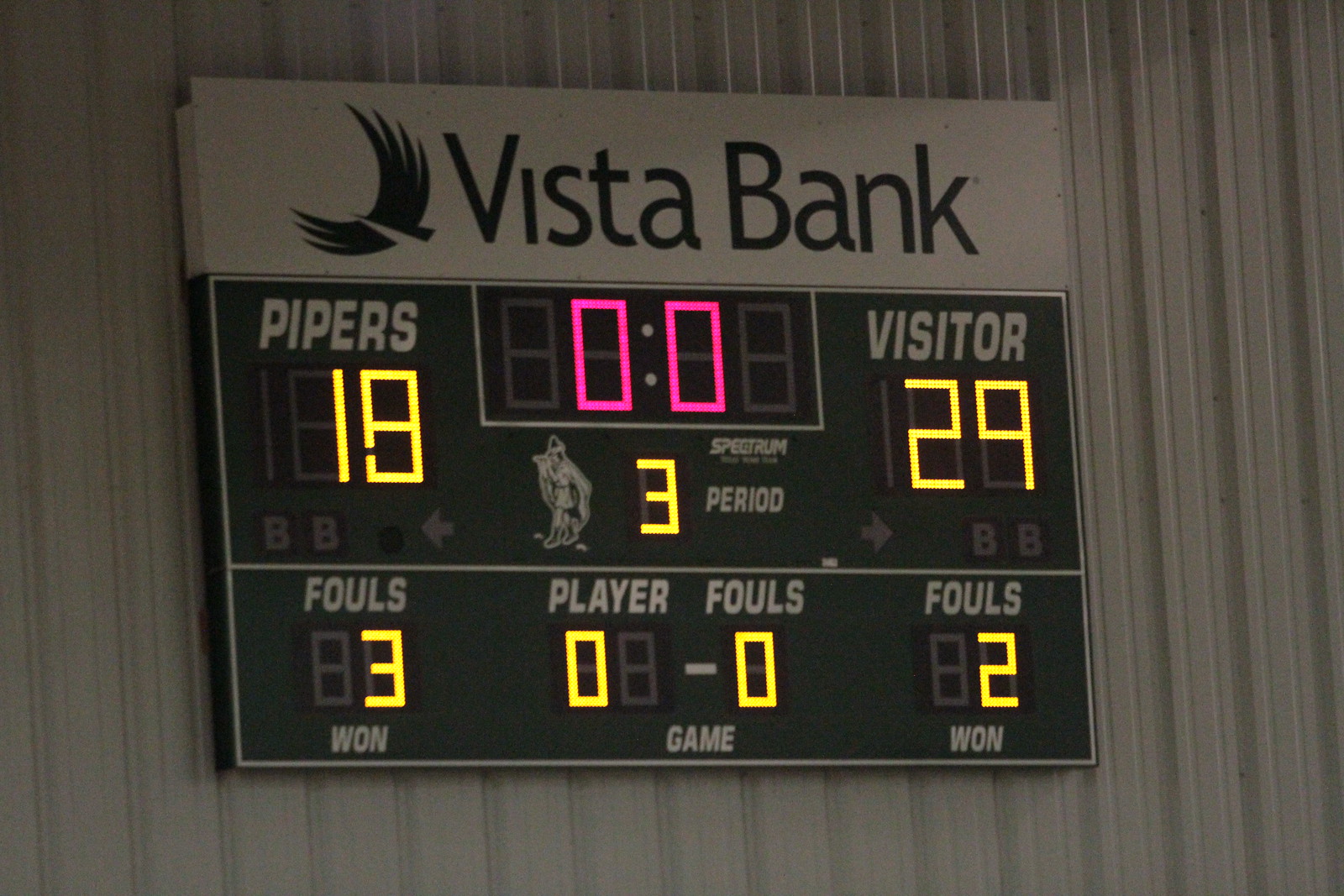The image features a color photograph of an electronic scoreboard mounted on what appears to be a backdrop of corrugated steel siding, which is gray. The scoreboard is divided into two sections: the top one-third is white and the bottom two-thirds is black. The white section at the top displays "Vista Bank" alongside an emblem of a winged bird, all in black lettering. Below this, the scoreboard transitions to a black background.

The central portion of the scoreboard prominently displays digital numerals. The team names “Pipers” and “Visitor” are illuminated in white, showing scores of 18 and 29 respectively. The period, indicated by a yellow-lit numeral, is the 3rd. The time clock, situated just below the team names, shows 0.0 in bright pink numbers.

At the bottom of the scoreboard, various categories are listed in white text: "Fouls," "Player," "Fouls," and "Fouls" again. Underneath these categories, specific numerals are lit in yellow. For the Pipers, the fouls stand at 3, the player number is 0, and the additional fouls show 0. For the Visitors, the fouls are indicated as 2.

The combination of bright yellow and pink digital numerals against the stark black and white sections creates a vivid, easily readable display, with the entire scoreboard affixed to a substantial-looking backdrop of corrugated metal.